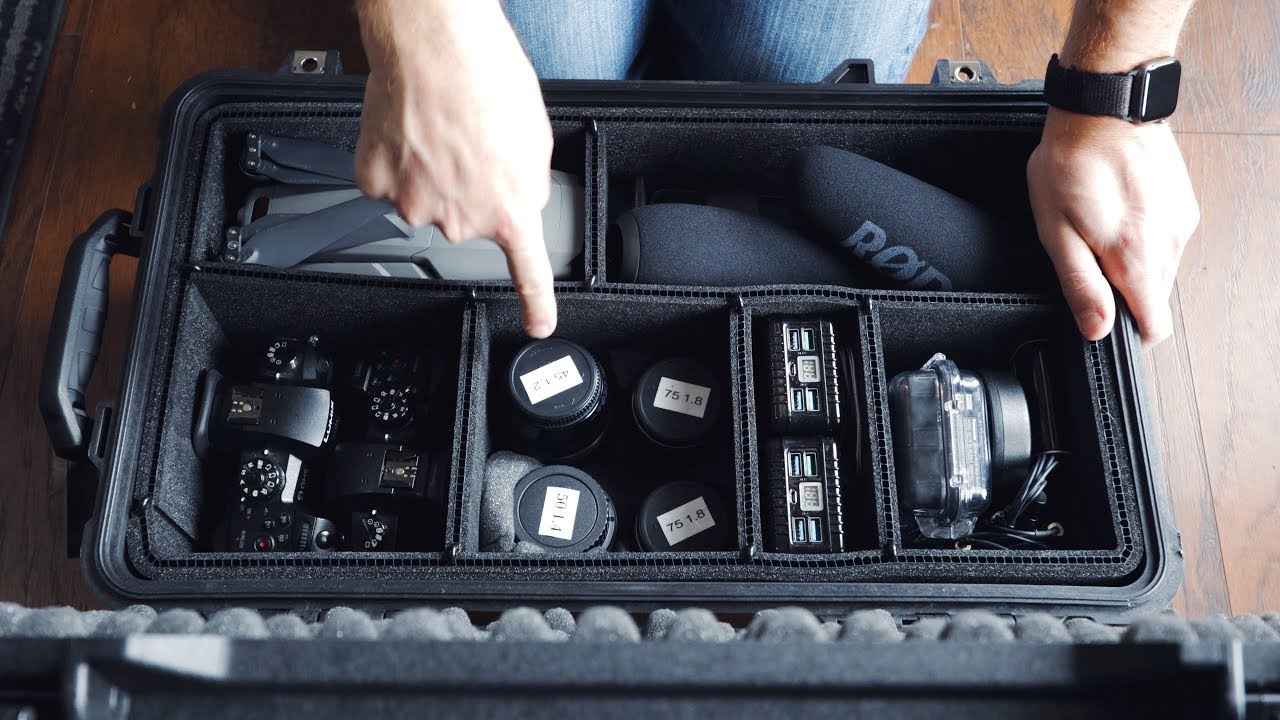The top-view photograph showcases a black, rectangular hard case designed for the protection and transport of camera equipment. It features six foam-padded compartments, providing robust protection for its contents. In the bottom compartments, there are two camera bodies of different models and four precisely labeled lenses: two 75mm f1.8, a 50mm f1.4, and a 45mm f1.2. The top right compartment houses a folded drone, while the adjacent compartments contain two microphones, chargers, and other accessories. The case also appears to have some specialized equipment and foam inserts, such as lens covers. Standing over the case, a man with blue jeans is visible from his thighs down, wearing a dark-banded smartwatch. He is kneeling on a brown hardwood floor pointing at one particular lens, emphasizing the meticulous organization of his gear.